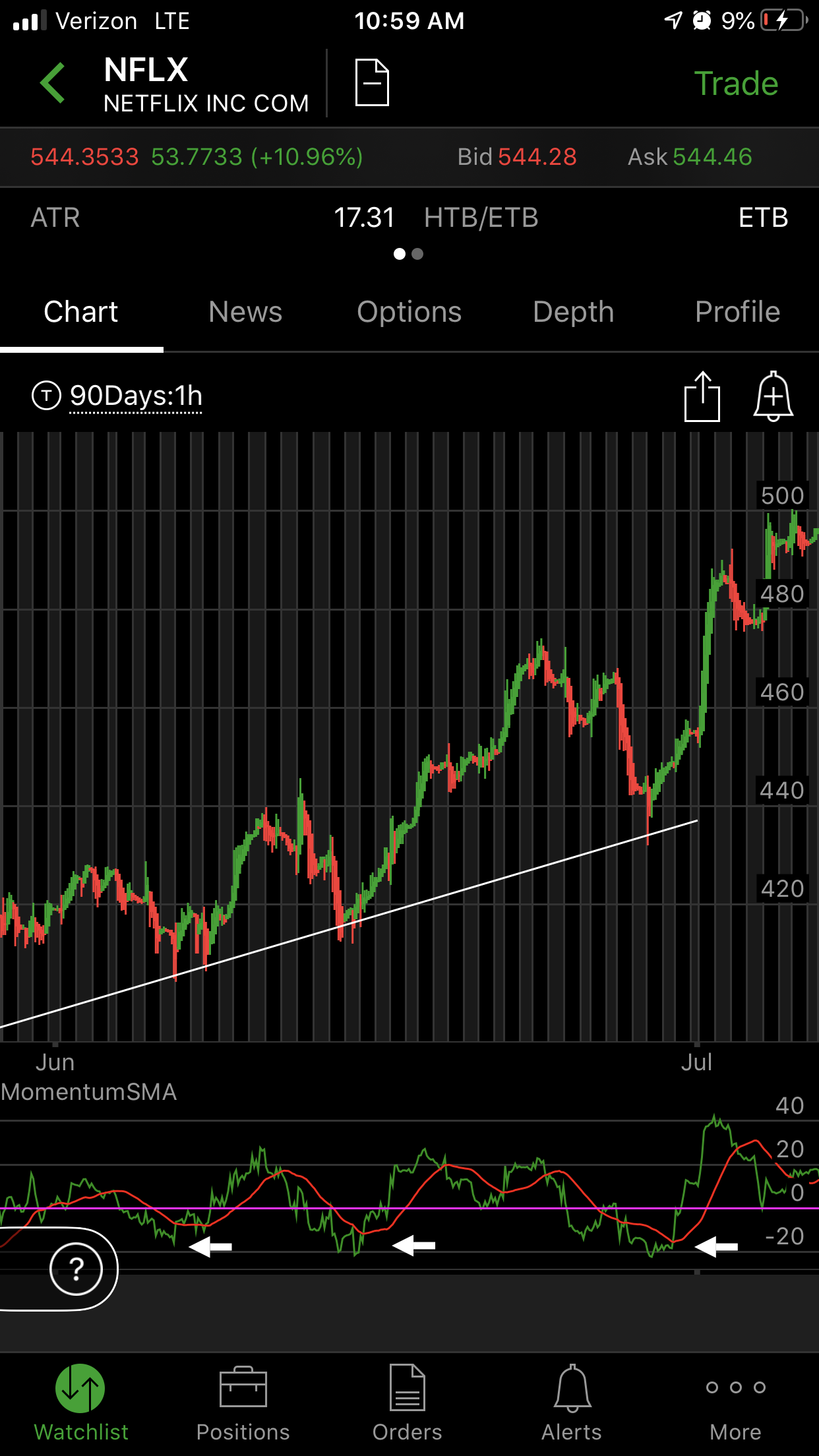Here's a detailed and cleaned-up caption for the image:

---

This screenshot, captured from a mobile device such as a phone or tablet, displays a detailed stock graph for Netflix (NFLX). The interface is set against a black background, typical of stock trading applications. 

In the top left corner of the screen, the Verizon LTE signal strength indicator shows three bars. The center of the header displays the current time as 10:59 AM, and the top right corner highlights a critically low battery level at 9%, alongside an active alarm icon.

Beneath the header, there is a green back arrow pointing to the left, followed by the stock ticker (NFLX) and the stock's full name, Netflix Inc. A "Trade" button, highlighted in green, is situated on the right side of this section.

There is a detailed breakdown of stock numbers below these labels. The most recent price appears in red at 544.3533, while the day's gain is displayed in green as 53.7733, with a percentage increase of +10.96%. The bid price in red is 544.28, and the ask price in green is 544.46.

Tabs labeled "Chart," "News," "Options," "Depth," and "Profile" are visible below the stock data, indicating different sections the user can navigate. 

The main graph shows the stock's performance over a 90-day period, with red and green lines plotting the price movements. The trend appears to be upward, with the price starting below 420 and nearing the 500 mark.

---

This caption provides a comprehensive and structured description of the screenshot's content, making it easy for readers to visualize the image.